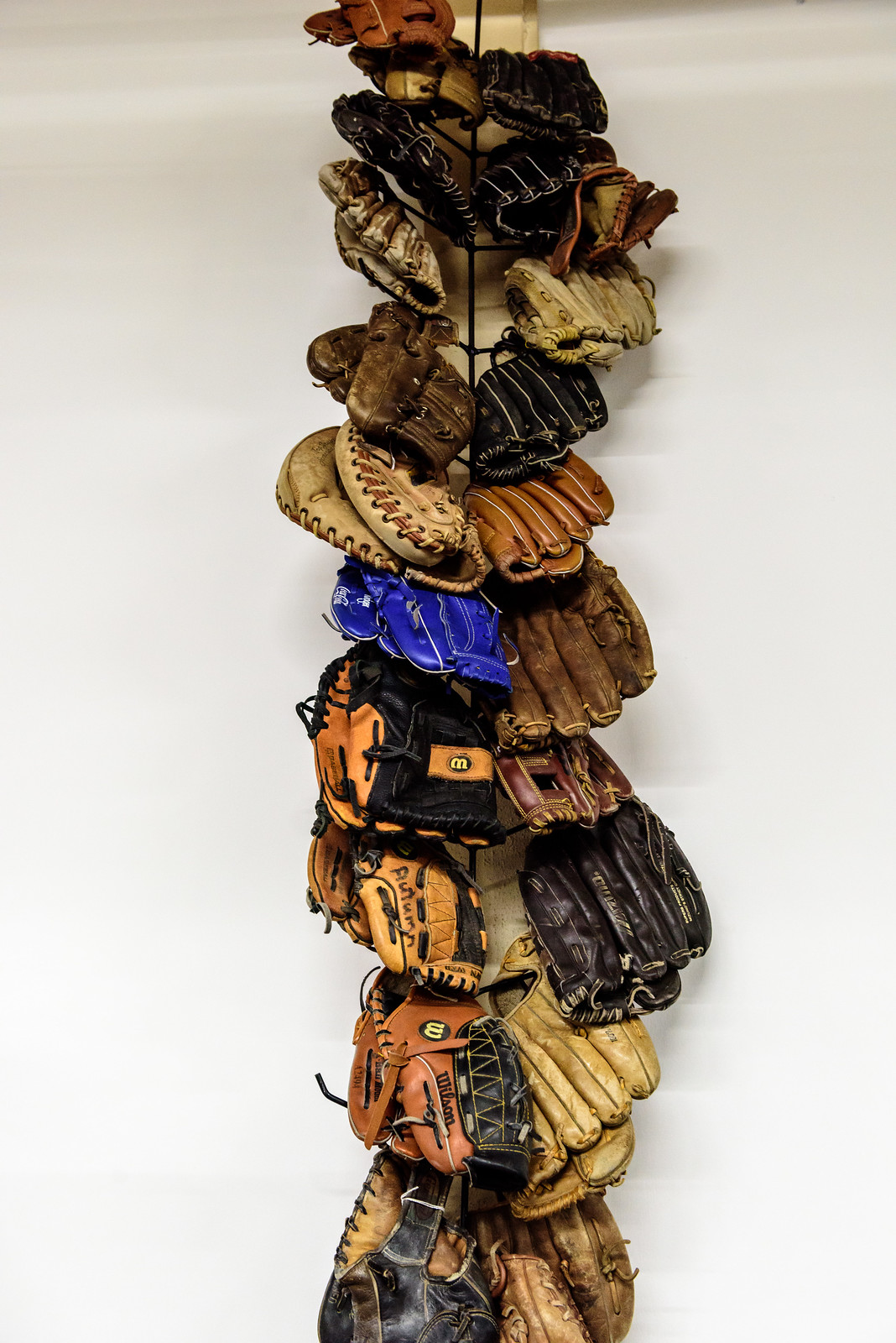This image features a unique, metal "tree" rack designed to hold an array of baseball gloves. The sturdy vertical metal structure stretches the entire height of the image, branching out horizontally to support multiple gloves. The background is a plain, unadorned white wall, casting soft shadows that add depth to the display. The gloves, in various states of wear, are arranged with the smaller, more worn ones near the top and progressively larger ones towards the bottom. The gloves showcase a spectrum of earth tones—ranging from light tans and dark browns to orange tans—with some distinctive exceptions, such as a bright plasticky blue glove. Specifically, from top to bottom on the left side, the gloves are brown (possibly gold), black, light brown, dark brown, tan, blue, and combinations of black with brown and brown with black details. On the right side, the sequence includes multiple black and brown gloves in various shades, an old ruddy brown, reddish brown, and finally a tan glove at the bottom. This inventive rack exemplifies a clever storage solution while highlighting the diversity of baseball gloves.